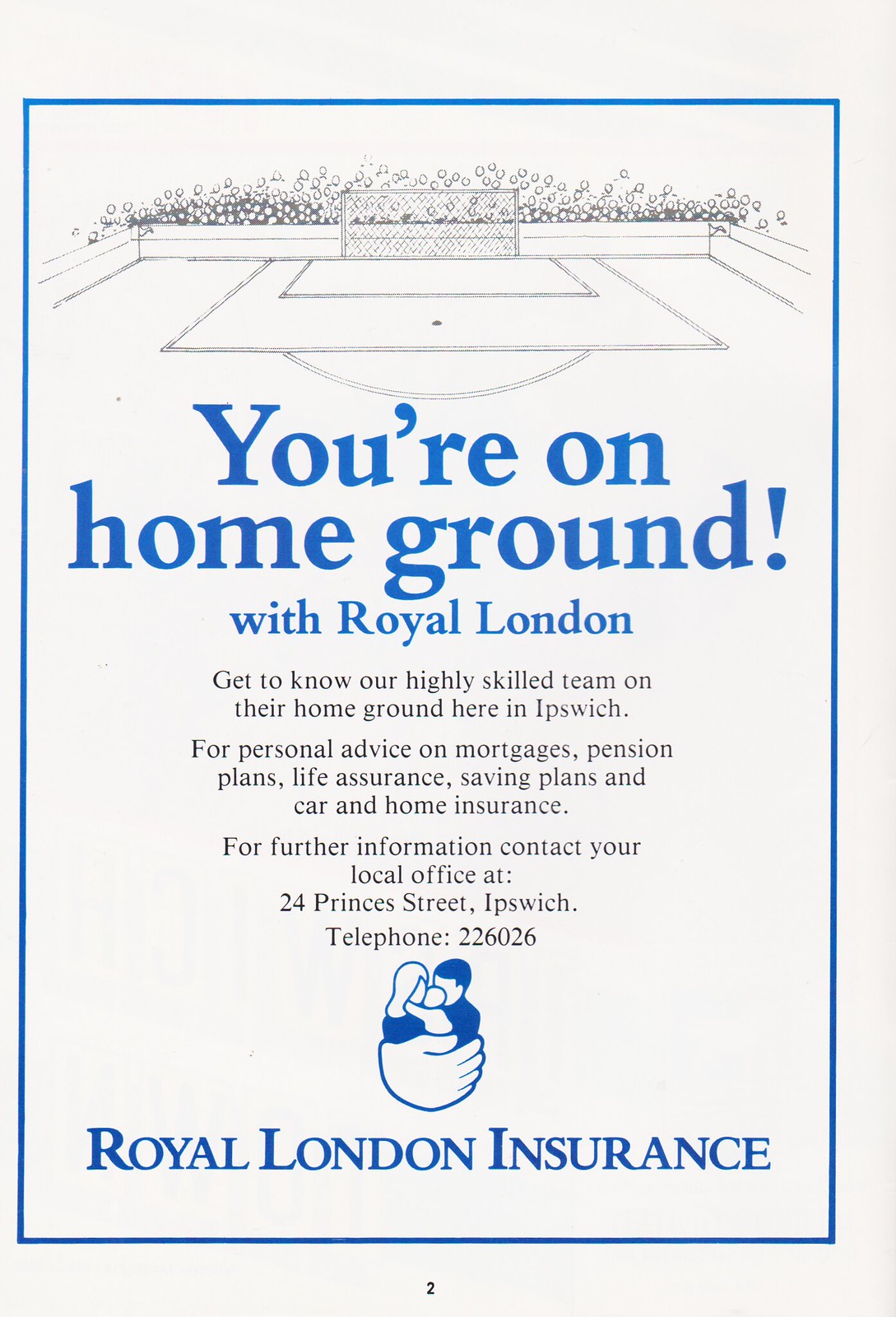The image is a vertical rectangular advertisement for Royal London Insurance, seemingly cut from a magazine. A prominent blue frame surrounds the content, with a detailed illustration of a section of a soccer pitch—showing the penalty box and goal—positioned at the top against a light gray and dark gray background. Below the illustration, in bold blue text, reads the headline, "Your Own Home Ground, with Royal London." This is followed by a block of black text that states, "Get to know our highly skilled team on their home ground here in Ipswich. For personal advice on mortgages, pension plans, life insurance, saving plans, and car and home insurance. For further information, contact your local office at 24 Princess Street, Ipswich, telephone 226026." Positioned beneath this text is the company logo, depicting a hand cradling a couple and a baby. The words "Royal London Insurance" are written in blue below the logo. The page number "2" is centered at the bottom of the ad. The page’s background has an off-white color that contrasts with the blue, black, and gray elements.